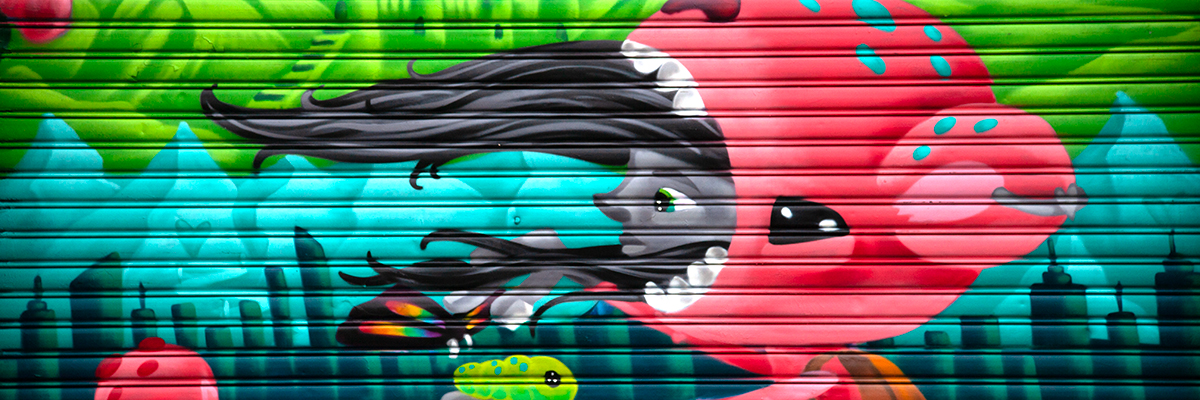This rectangular image, oriented with its long side from left to right, vividly captures a surreal scene. Dominating the center is an extraordinary creature with its mouth agape, revealing stark white teeth. The creature’s body is primarily reddish, adorned with a pattern of blue circles or dots, and it has eyes positioned on the sides of its head. Emerging from the creature's open mouth is a human-like face with greenish eyes and gray skin. Wisps of nearly black hair flow out from the mouth, framing the face above and below.

In the background, a cluster of buildings in a cityscape are faintly visible, rendered in dark green hues. Beyond the city lie mountains, which transition into a teal color, and above them, the sky shifts to a definite green tone. On the left side of the image, there are two to three other fantastical creatures, bearing red and green colors, adding to the image's otherworldly charm. This intricate composition combines elements of fantasy and reality, creating a strikingly detailed and imaginative scene.